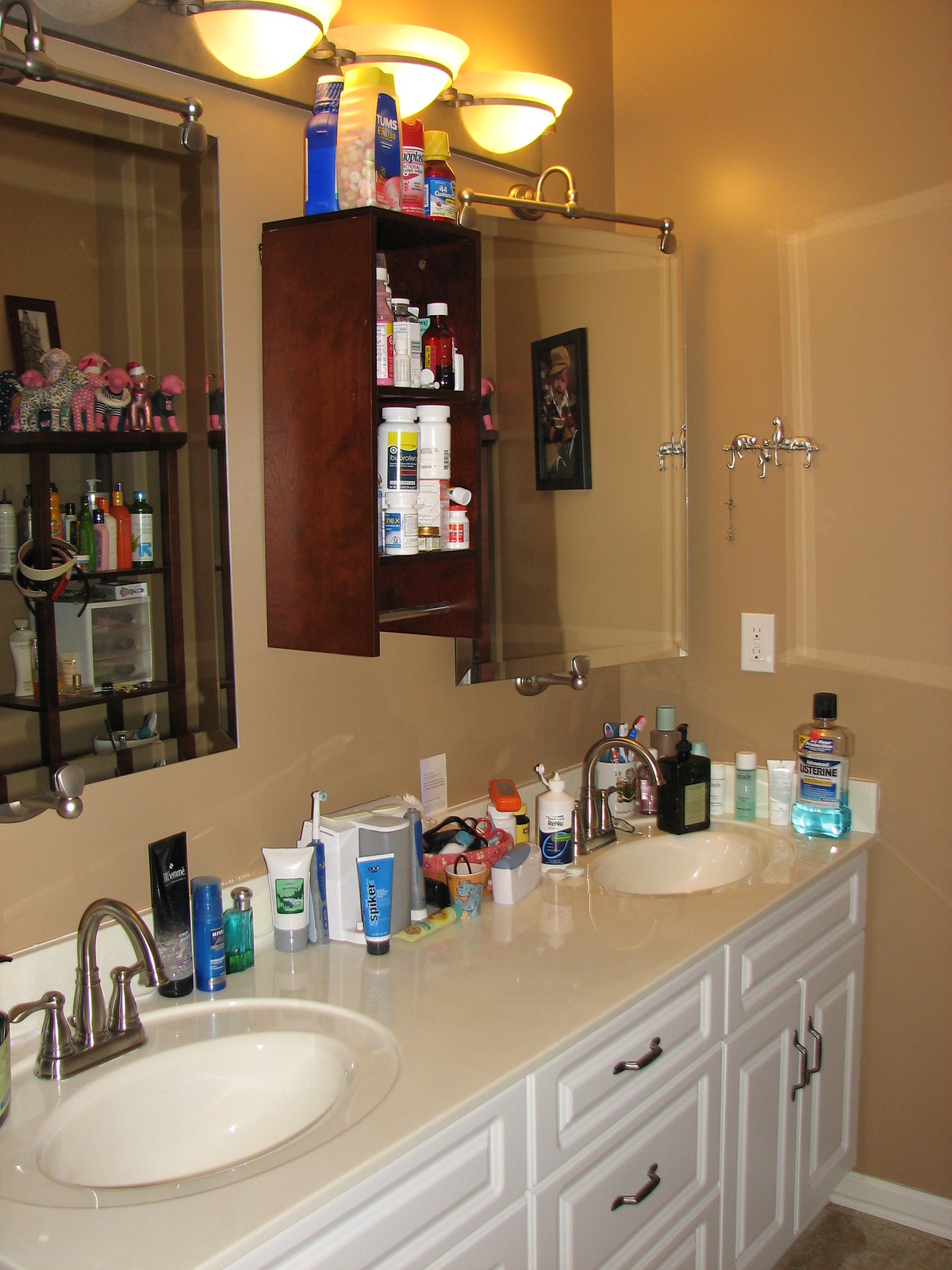The image showcases the interior of a bathroom characterized by twin sinks. The countertop is cluttered with various cosmetics. Beneath the sinks are white drawers and cabinets. Above each sink, there are mirrors and vanity setups. The mirror on the far right reflects a picture of a baby. Adjacent to this mirror is a small brown shelf affixed to the wall, filled with and topped with assorted medications.

Another mirror is positioned nearby, reflecting a shelf adorned with small toy dog sculptures, some of which are pink, including a Dalmatian. The lower shelf holds additional cosmetic items while another tier contains a small box or container filled with miscellaneous items. The entire setup is illuminated by a warm, yellow light positioned above the mirrors and shelf.